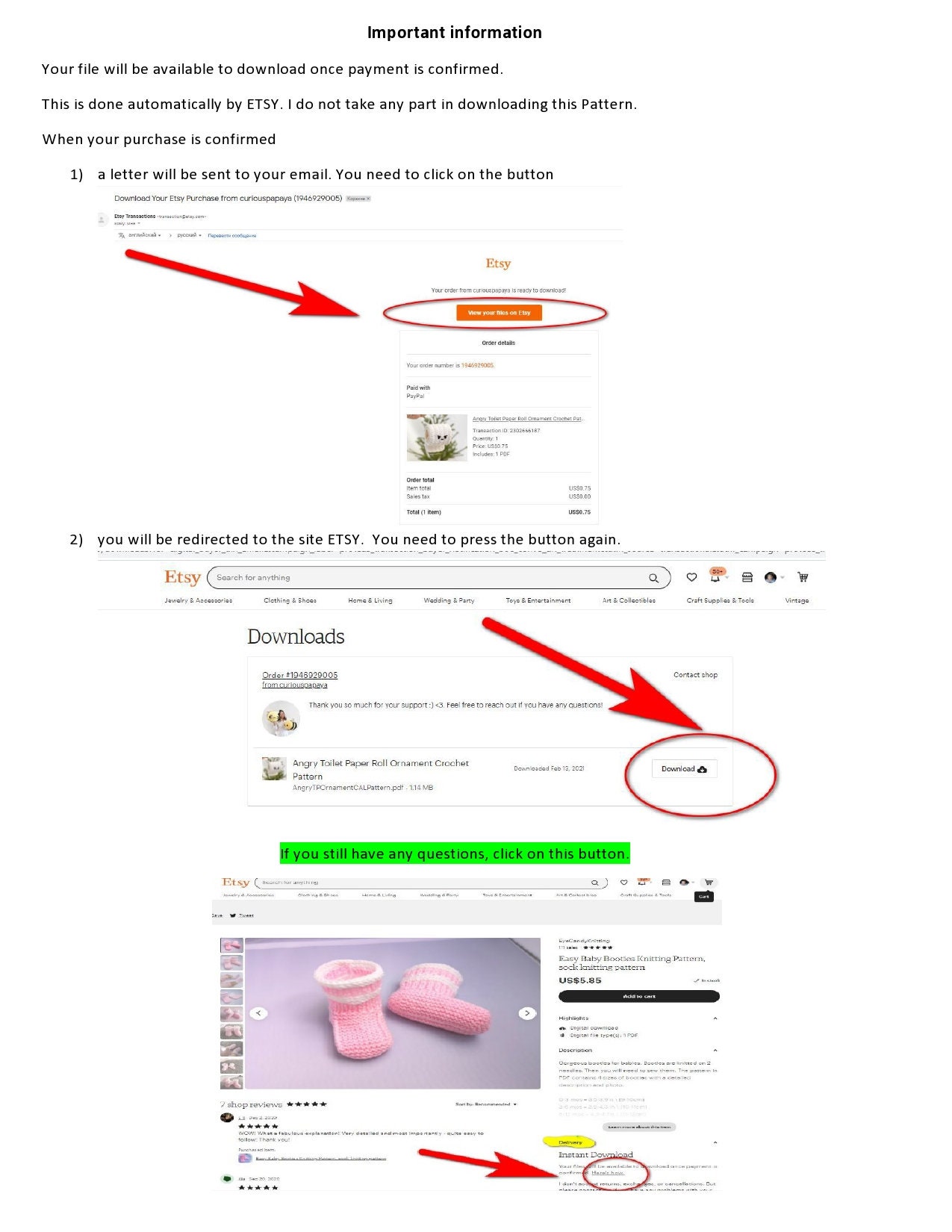This image appears to be a step-by-step guide on how to download a purchased pattern from Etsy after payment confirmation. At the top, there is a section titled "Important Information." The guide states that the file will automatically become available for download once payment is confirmed, a process managed by Etsy without the seller's involvement.

The first step, labeled "1," shows an email that will be sent to the buyer after purchase confirmation. This email contains an orange button, circled in the image with a big red arrow pointing to it. The button says "View your files on Etsy." 

The second step, labeled "2," indicates that clicking this button will redirect you to an Etsy page. On this page, another download area is highlighted, again with a big red arrow. This area contains an icon where the pattern file can be downloaded.

At the bottom of the image, in the right-hand corner, there is additional information for users who still have questions. It points to a button with instructions, directing them on where to click for further assistance. 

The visual guide effectively uses arrows and highlights to clarify the steps for downloading the purchased pattern.